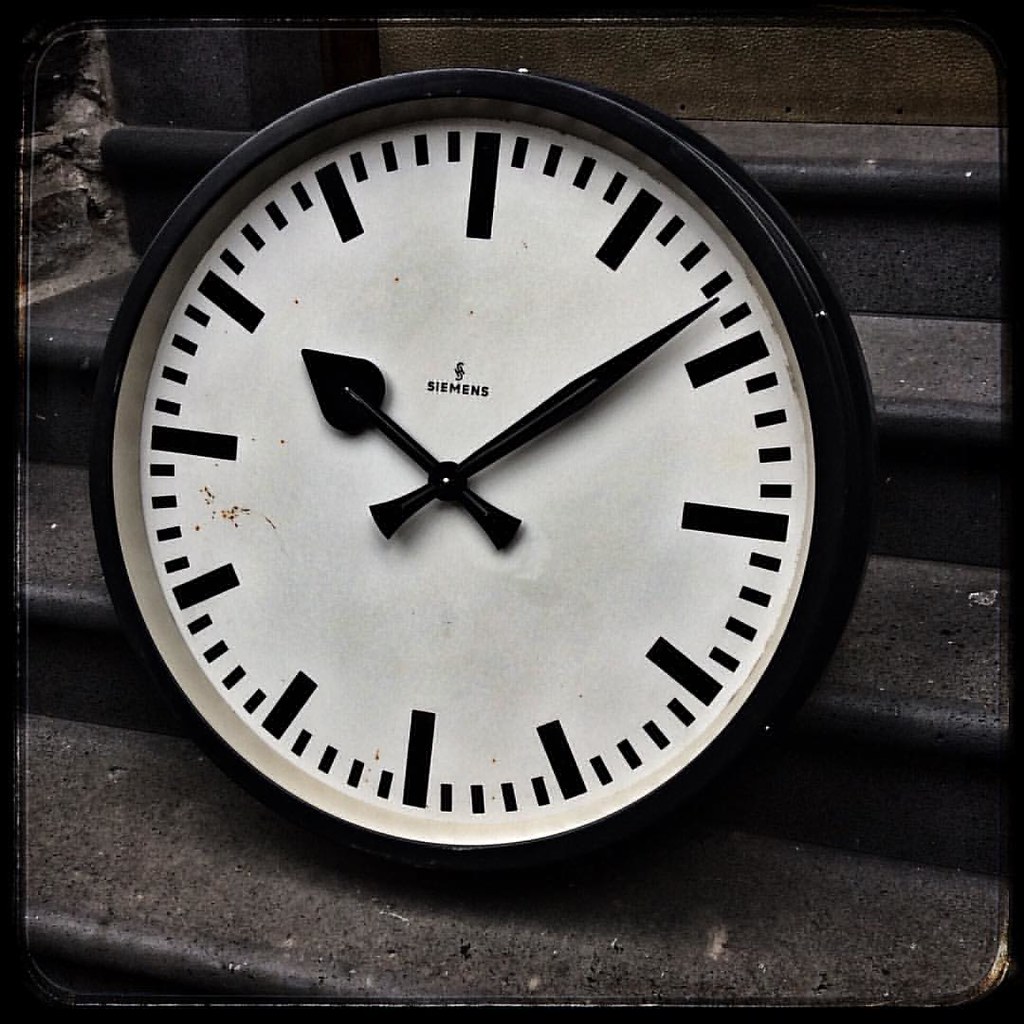In the image, a gray staircase with multiple steps ascends and descends, creating a dynamic pathway. At the center of this scene stands a prominently featured clock. The clock bears the name "Siemens" displayed across its front. The clock's hour hand points towards the 10th rectangular marker, while the minute hand rests between the 1st and 2nd markers. Surrounding the clock face are numerous small dash marks interspersed between larger rectangle markers. The clock face itself shows signs of wear and grime, particularly noticeable on the left side near the hour hand. The entire image is rendered in a monotone palette, characterized by dull and muted colors, with subtle shading adding depth and a slightly weathered appearance to the scene.